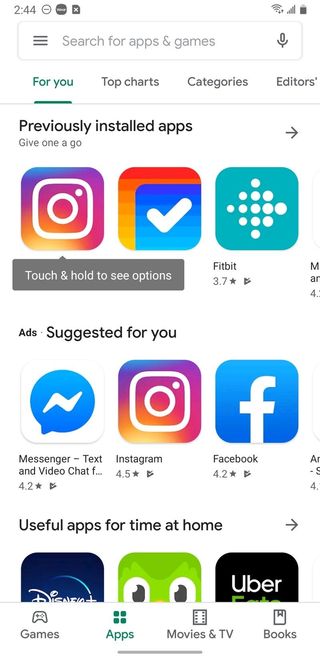This screenshot captures the Google Play Store interface on a mobile device. At the top, a search bar reads "Search for apps & games" and is accompanied by a microphone icon for voice search on its right. Below the search bar are four navigational tabs: "For you" (selected), "Top charts," "Categories," and "Editor's choice." 

The main content is organized into several sections, starting with "Previously installed apps," which shows the icons for Instagram and Fitbit, though a third app is obscured. Next is "Ads suggested for you," featuring Facebook, Messenger, Instagram, and Facebook again, each with star ratings: Messenger (4.2 stars), Instagram (4.5 stars), Facebook (4.2 stars), and Fitbit (3.7 stars). 

Further down is the "Useful apps for time at home" section, listing Disney+, a VR-related app, and Uber Eats. At the very bottom of the screen, there are tabs for "Games," "Apps," "Movies & TV," and "Books," with "Apps" currently selected. 

The interface sports a clean, white background with colorful text icons and follows Google's sleek, modern design aesthetic.